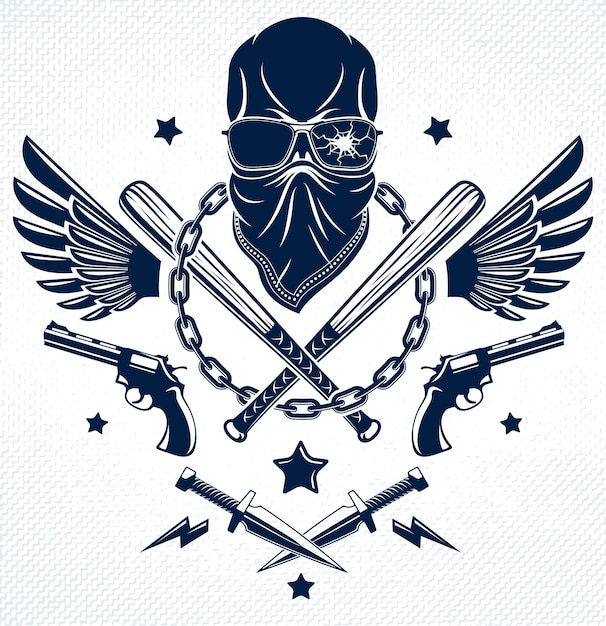A square image with a subtle diagonal zigzag pattern in the background, featuring light gray lines on white, gives a textured appearance. At the center is a dark blue, helmet-like head with detailed, white-rimmed glasses—one cracked with crooked white lines. The figure wears a blue bandana with a white dotted pattern around the neck. Bird-like wings extend from where the arms would be, with two crisscrossed baseball bats at the center of the body area encircled by a large silver chain. Beneath the wings are handguns pointing outward, and at the bottom are two swords forming a cross. Scattered around are navy lightning strikes and stars.